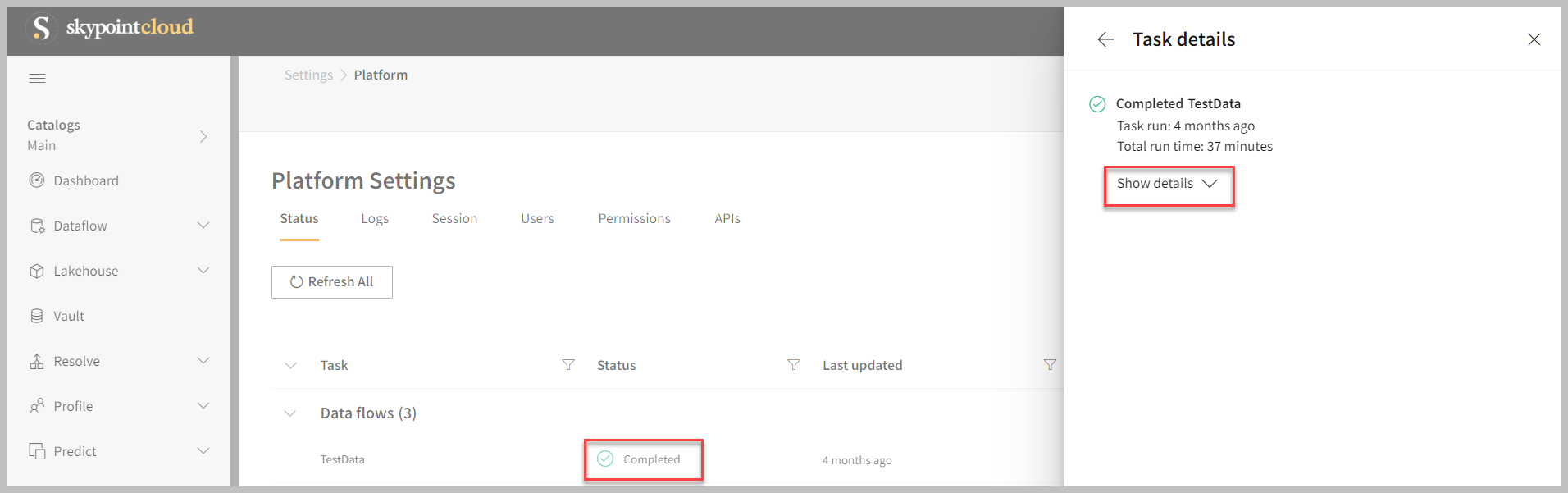The image depicts a detailed user interface of a data management platform, prominently featuring various navigation elements and status indicators. The layout includes:

1. **Top Navigation Bar**:
   - **Hamburger Icon**: Likely for accessing a side menu.
   - **Categories**: Broad sections within the platform.
   - **Main Dashboard**: Central hub displaying key information and metrics.
   - **Date Flow**: Presumably for tracking data transitions over time.
   - **Lake House**: Possibly a data lake interface.
   - **Vault**: Secure data storage section.
   - **Resize**: Option to adjust the UI layout.
   - **Profile**: User account settings.
   - **Predict**: Analytics or forecasting features.
   - **Settings**: General platform configurations.

2. **Main Dashboard Section**:
   - **Status**: Underlined in orange, indicates the platform's current operational state.
   - **Logs**: Record of system activities and events.
   - **Session**: Information on active sessions.
   - **Users**: Management of users within the platform.
   - **Permissions**: Control over user access rights.
   - **APIs**: Interface for application programming interaction.
   - **Refresh All Tasks**: Option to update or reload tasks.
   - **Status**: Additional status indicator with the note **Last Updated**.
   - **Data Flows (3)**: Indicates three data flow tasks.

3. **Task Quota and Status**:
   - **Completed**: Highlighted with a green circle and green check mark. Surrounded by a red rectangle, indicating special attention or notification.
   - **Four months ago**: Date of completion indication, noted in parentheses.
   - **Task Details**: Actionable items with a left arrow and an X icon for navigation and closing.
   - **Completed Test Data**: Specific data set completion status.

4. **Run Details**:
   - **Task Run Four Months Ago**: Time since the last task execution.
   - **Total Run Time**: 37 minutes specified.
   - **Show Details**: Red rectangle highlighting this option for viewing more detailed information.

Every element builds a comprehensive view of the system's functionality, recent activities, and user options, ensuring users can seamlessly navigate, monitor, and manage the data platform efficiently.